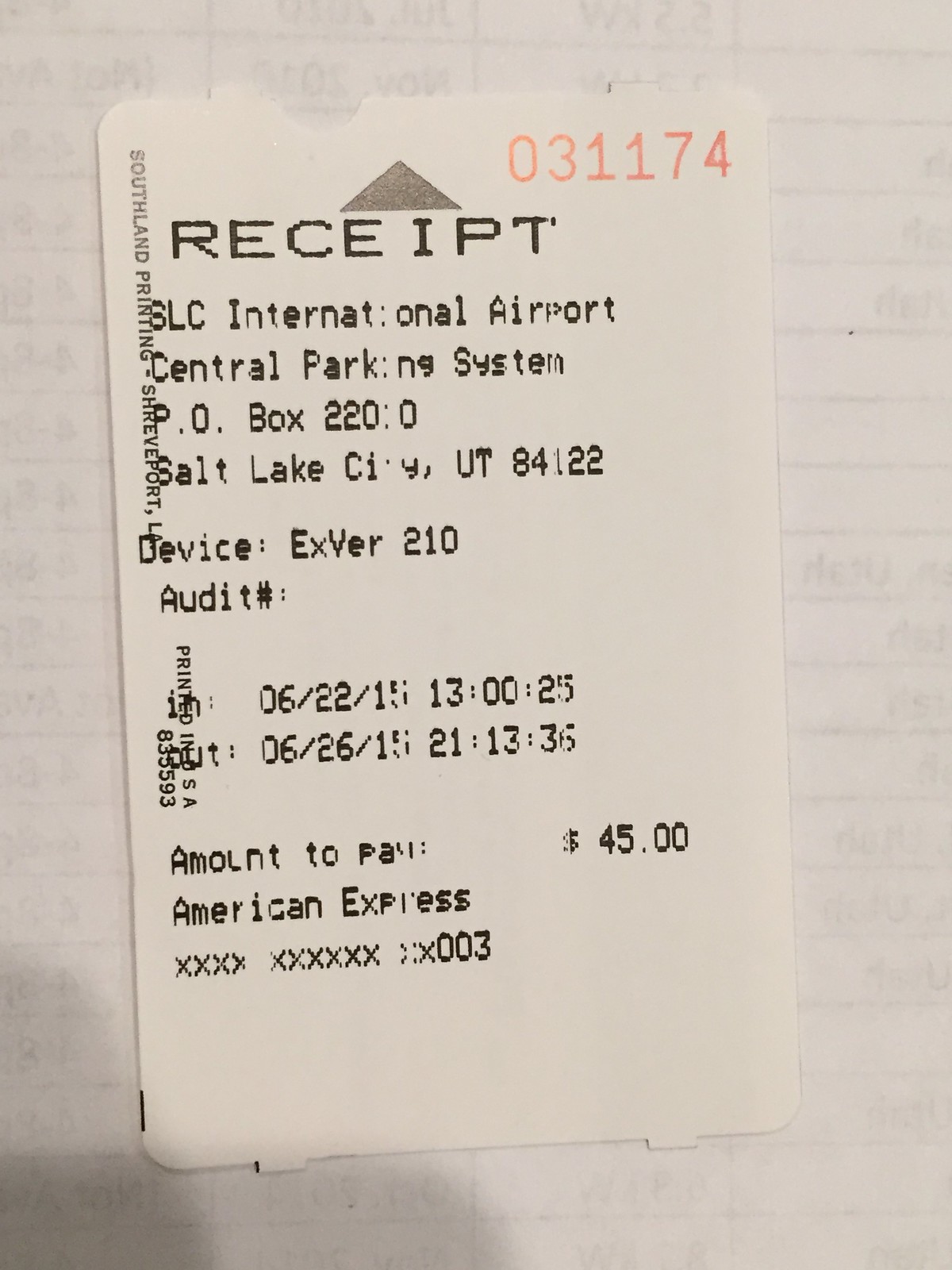The image depicts a white paper background cluttered with various squares, rectangles, and text fragments, which appear slightly out of focus and not easily legible. In the top right corner, there is a clear imprint of the number "031174". Near this number, a gray triangle points upward. The text content on the document resembles details typically found on a receipt. The detailed information suggests a connection to the SLC International Airport's Central Parking System:

- Address: PO Box 220, Salt Lake City, Utah, 84122
- Device: X0210
- Audit Number: 835593
- Printed in USA
- Print Date: 06-22-15, 13:00:25
- Usage Period: 06-26-15, 21:13:36

The image also states the amount to be paid, which is $45, and a partially obscured American Express credit card number ending in 0003.